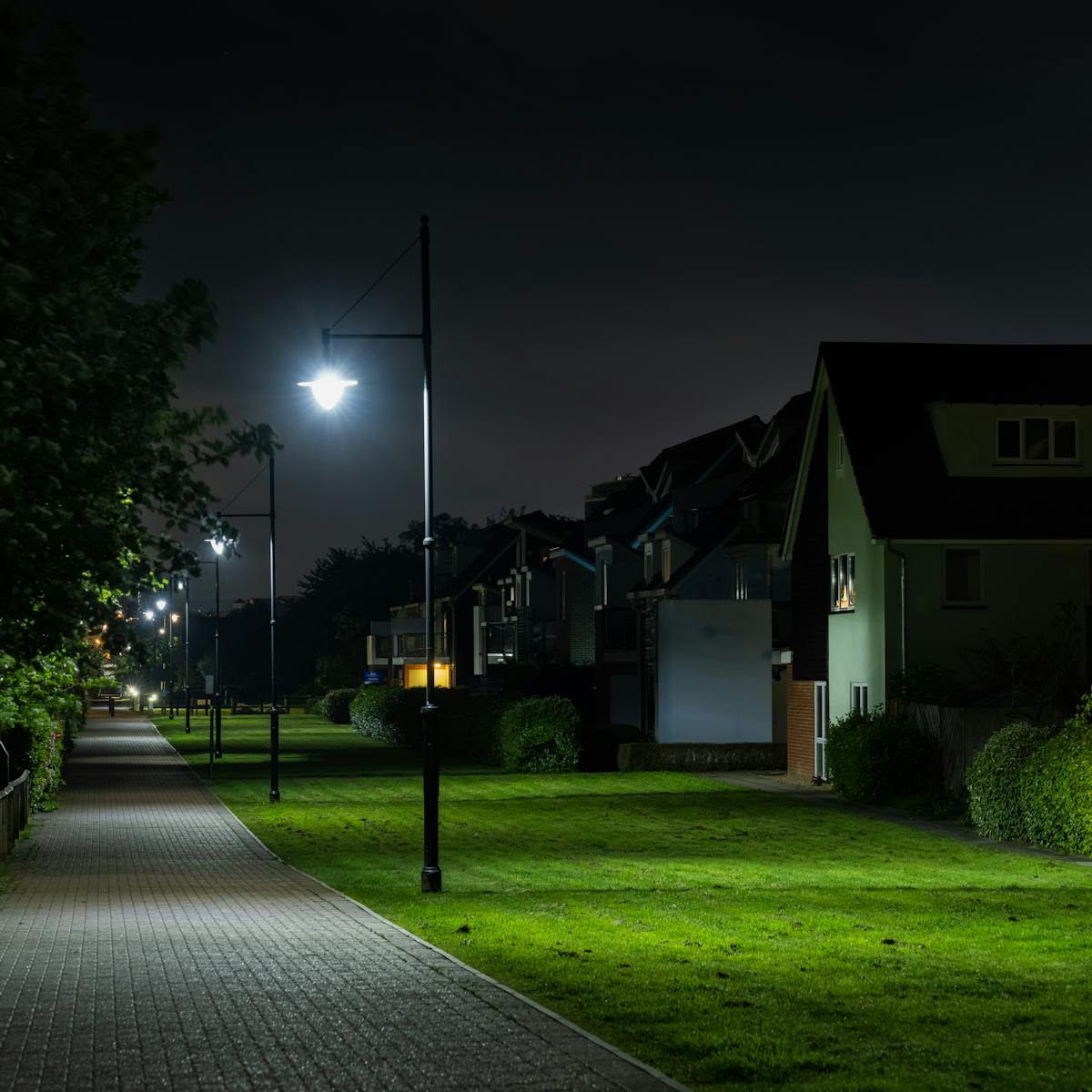This square color photograph, taken at night, captures a suburban neighborhood scene from a brick-paved sidewalk. The camera, positioned on the left side of the sidewalk, faces down its length, revealing well-maintained lawns and backyards of row houses on the right. The area is lined with tall lampposts, each illuminating neatly mowed grass and perfectly trimmed bushes. The scene is distinctly peaceful, with the dark sky overhead enhancing the glow of the streetlights and the occasional bright orange porch light in the distance. The landscape is flat with trees silhouetted against the black sky. In the distance, a lone figure can be seen walking down the sidewalk, adding a human element to this serene neighborhood setting. The photograph, devoid of any road, focuses solely on the walkway, lawns, and the subtly illuminated homesteads, highlighting the unique layout of this middle-class, neatly planned community.